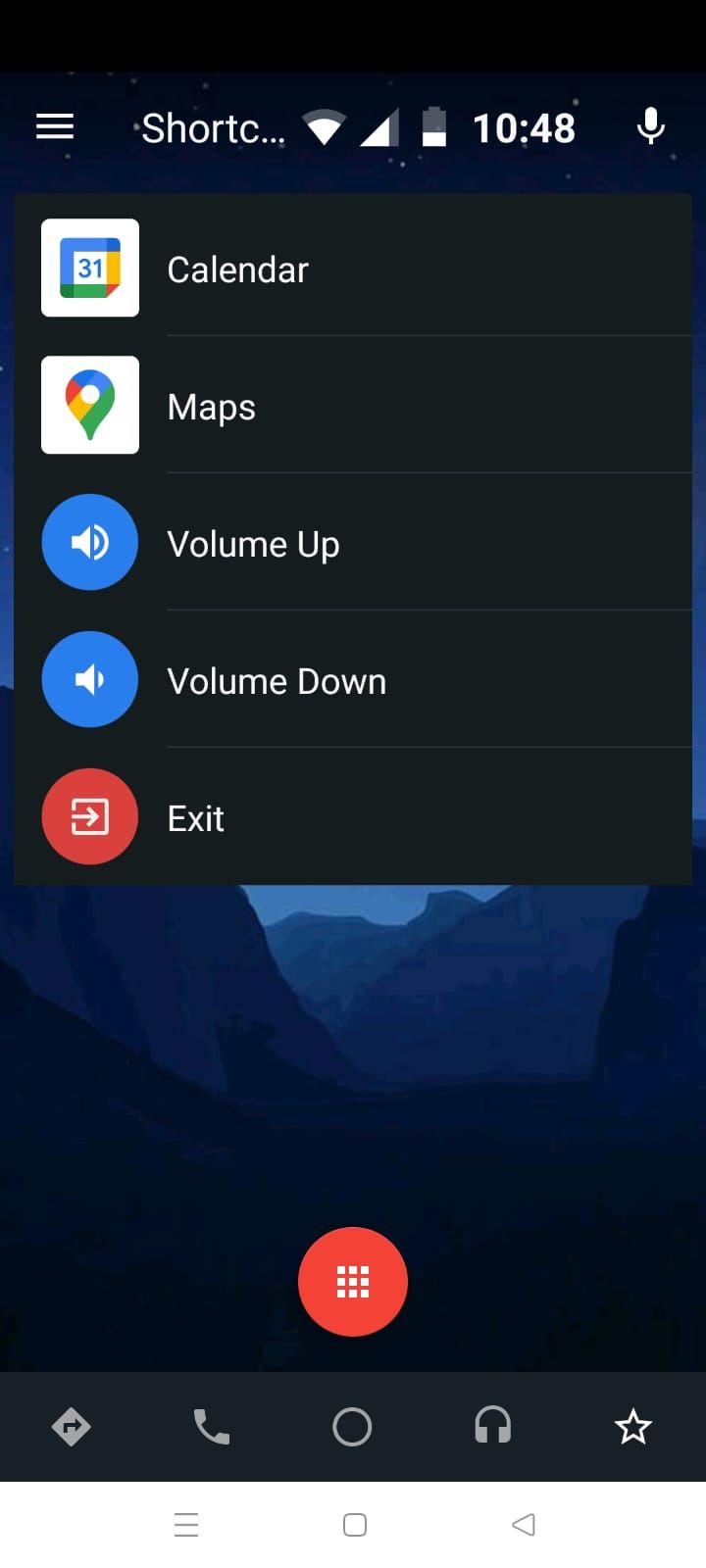The image displays the interface of a smartphone screen with a completely black background. At the top left corner, there is a white triple-stacked line menu icon indicating a navigation menu. Next to it, partially visible text reads "SHORTC...," likely an abbreviation for "Shortcuts." 

On the same top row, the right side shows the Wi-Fi signal bar and a battery icon that appears to be nearly empty, indicating a low battery. The time is displayed as 10:48. To the far right, there's a microphone icon suggesting the option to initiate a voice search.

The main section of the screen features several app icons and text labels, arranged in a vertical list. The first icon is the Google Calendar, represented by a small calendar graphic with the label "Calendar" beside it. Just below this, the Google Maps app is shown with an upside-down teardrop icon, commonly used for location pins, labeled as "Maps."

Further down, there are two blue circle icons for volume control. The first blue circle has a speaker icon and is labeled "Volume Up," while the second, smaller speaker icon immediately below it is labeled "Volume Down." 

Following these, a red circle contains a right-pointing white arrow on a white square, labeled "Exit." Beneath this, there is a dim graphic that resembles a mountainous landscape under a blue sky, but it is faint and hard to discern clearly.

Continuing down, another red circle features a grid of nine white dots arranged in three rows and three columns, reminiscent of a miniaturized face of a Rubik's Cube.

At the very bottom of the screen lie the standard smartphone action icons: a share icon, a phone headset icon, a circle-shaped icon for exiting or returning to the home screen, a headphone icon, and a star icon typically used for favorites.

The overall image provides a detailed snapshot of a smartphone's user interface with specific icons and functions prominently displayed against a stark black background.